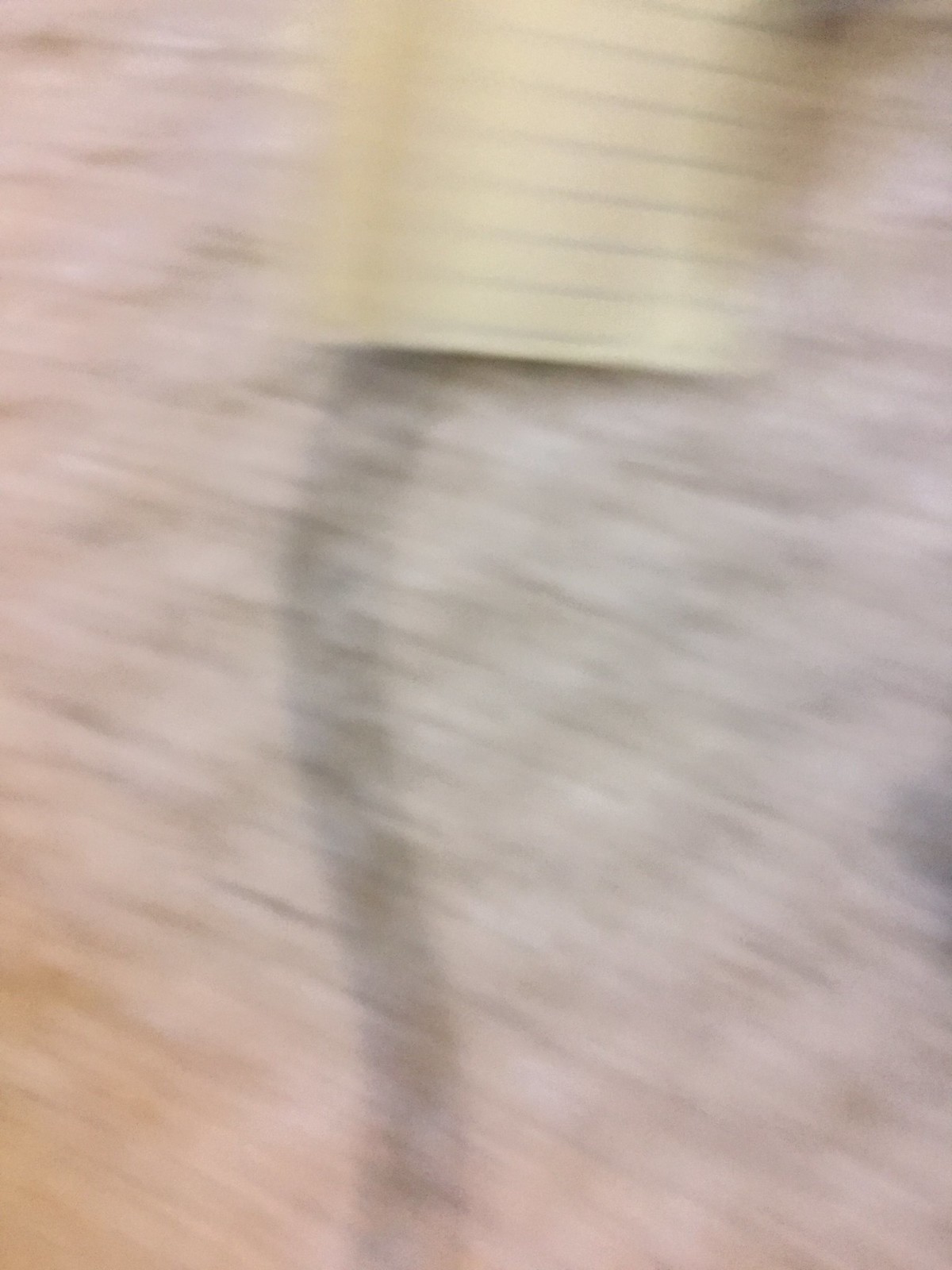This image is a large, rectangular photograph characterized by extreme blurriness indicative of motion, likely due to shaky hands during capture. The dominant hues are shades of peach, light tan, gray, and white, with splashes of yellow and pink. The photo features a distinct, slightly curving thick black line that stretches horizontally across the middle, resembling a shadow or possibly a cat's tail. Along the top, there appears to be a piece of lined, yellow paper with blue horizontal lines, though the severe blurriness makes it challenging to discern. The background texture suggests a variegated pattern, resembling a gray and white carpet, with motion lines angling from the top left to the bottom right. The overall visual impression is one of chaotic yet dynamic movement, with no distinct forms or shapes but an overwhelming sense of speed and motion.